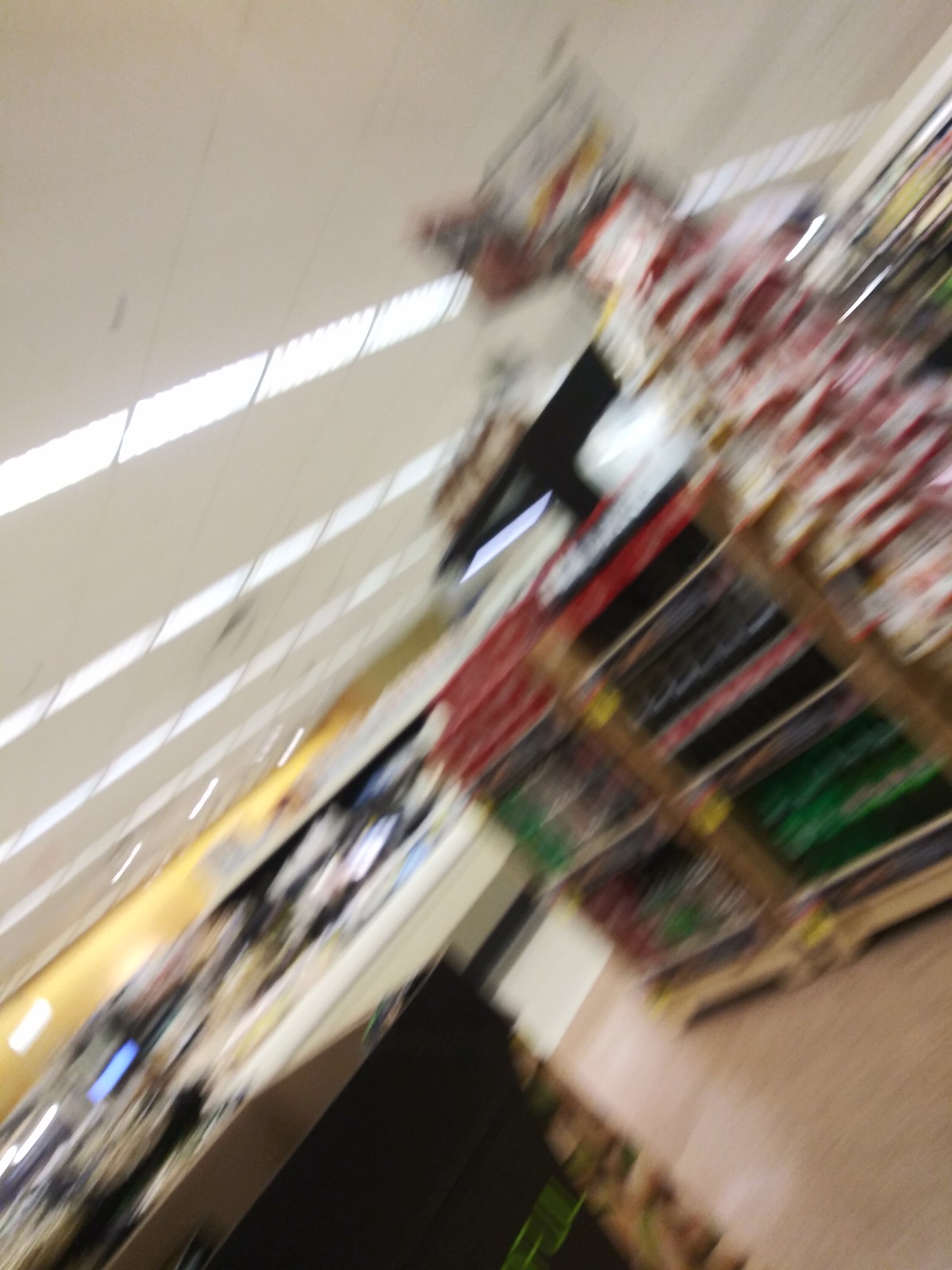This image, despite being blurry and distorted due to a moving camera, depicts the interior of a grocery store, likely at the register area. The ceiling, visible in the top left corner, features recessed fluorescent lighting and white ceiling panels. Below, there are shelves and coolers along the aisles. Notably, a fridge at the register area contains two-liter soda bottles, including brands like Coca-Cola, Diet Coke, Mountain Dew, and green Sprite bottles. On the right, a shelf displays more soda bottles. Additionally, there is a container on the left likely filled with nuts. Behind the register area, a yellow wall and a larger frozen fridge section can be seen. The ground has tiled flooring and the entire store is well-lit, neatly organized, and stocked with various items, despite the image's out-of-focus quality.